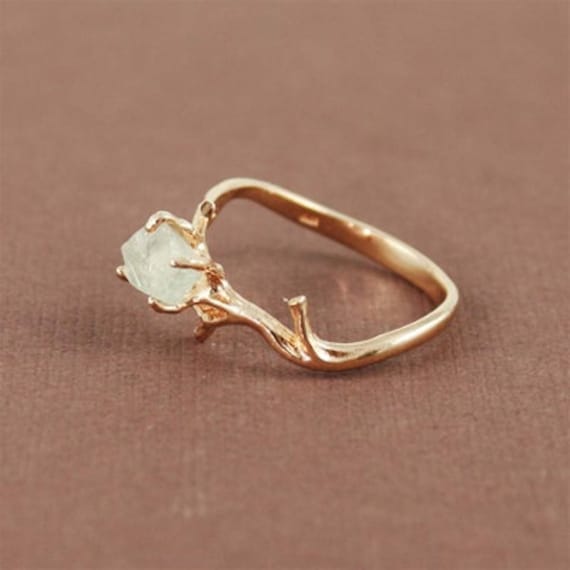The photograph appears to be a professional catalog image showcasing a stunningly unique, handcrafted engagement ring. The ring itself is made of what looks to be real gold, although its exact karat and purity are indiscernible due to the small stamp on the inside of the band which is too tiny to read clearly. The design of the ring is highly distinctive, featuring a twig-like shape that accentuates its naturalistic aesthetic. The band is slightly thicker at the back, tapering towards the front where it splits into delicate, branch-like extensions.

These branches form prongs that cradle a faceted, non-transparent stone. The exact type of the stone is uncertain; it could either be an unusually cut diamond or perhaps a piece of quartz. The prongs holding the stone are particularly notable for their remarkable resemblance to slender, elongated fingers, further enhancing the organic, artisanal craftsmanship of the piece. Along the front of the ring near the prong settings, there is a textured, striated bark-like pattern that emphasizes the twig and branch motif.

The ring is displayed against a sophisticated backdrop, which appears to be the lid of a brown, faux leather jewelry box, adding a touch of elegance and highlighting the refined artistry of this exceptional piece.